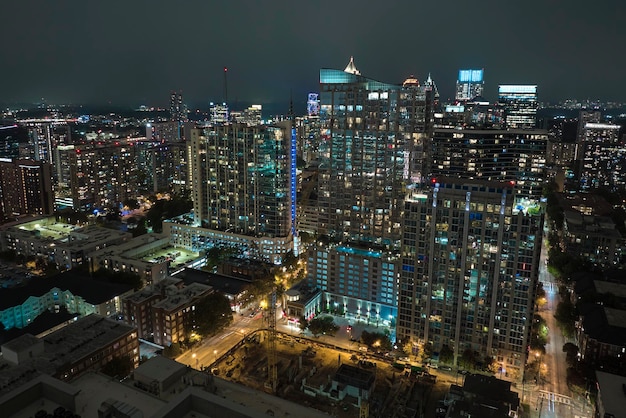The horizontal color photograph captures a nighttime cityscape featuring an expansive range of building heights, spanning from six storeys to towering skyscrapers 20 to 40 storeys high. The city is vibrantly lit, with about half of the windows illuminated by various colors, including blue, yellow, gold, green, and white. The scene encompasses approximately six to seven city blocks, giving an impression of a dense urban area, likely a downtown zone of a major or semi-major city. The streets below are sporadically lit by streetlights and punctuated with a few vehicles and pedestrians. Trees and pockets of greenery intersperse the street level, adding a touch of nature amid the urban environment. The sky is dark and cloud-filled, with fog visible in the distance, and a notable large tower with a red light on its antenna punctuates the background, adding a distinctive element to the cityscape.